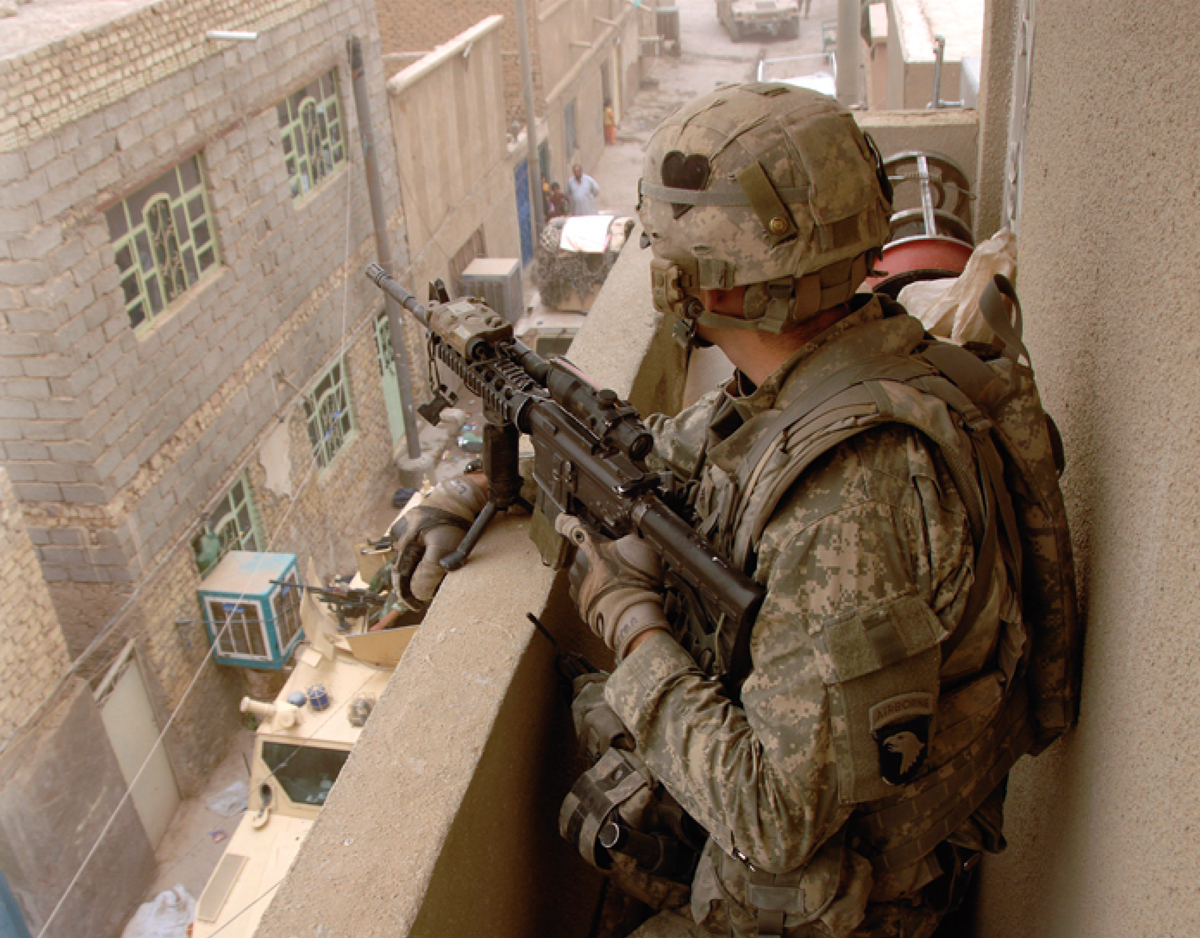In this color photograph, we see a U.S. soldier in full tactical gear standing on a narrow, chest-high cement balcony. The soldier is wearing Desert Storm camouflage from helmet to knees, which includes a helmet with a distinctive brown heart patch and an "Airborne" patch with an eagle on his shoulder. He holds a black rifle in his left hand while his right hand rests over the balcony rail. The soldier is turned slightly to the side, looking down into a narrow, dusty alleyway.

Below, the scene captures what looks like a Middle Eastern urban landscape. The alley is flanked by a row of sand-colored, worn-down buildings with concrete and stone facades, some of which have green frames around the windows and occasional air conditioners. On the ground, multiple tan military vehicles—including Humvees—are parked, and several people, including a man in a blue shirt and a small child in a red shirt, are seen walking. The alleyway appears to stretch into the distance, with a tan military truck and another vehicle just entering the frame. The overall image has a slight haze, suggesting the presence of a sandy dust typical of desert conditions. The soldier appears vigilant, embodying a scene that captures the tensions of a combat zone.